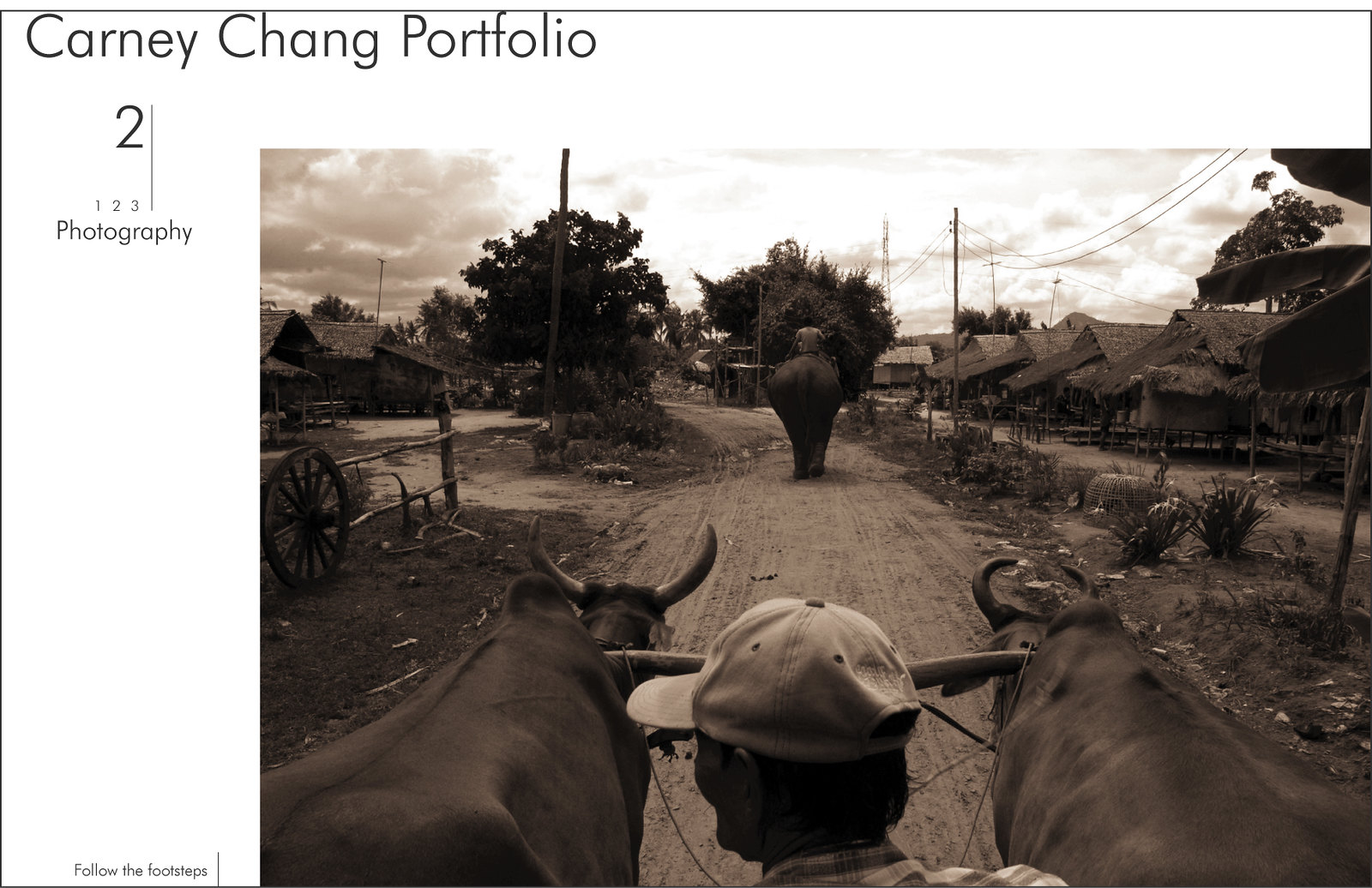This sepia-toned photograph, framed by a white border on the top and left, showcases a rustic village scene with an old-world charm. The top left of the border bears the title "Carney Chang Portfolio" followed by "2123 Photography," while the bottom left corner reads "Follow the Footsteps." The photograph itself captures a dirt road winding through the village, lined with hut-style buildings and trees on both sides. In the foreground, two oxen are yoked together, pulling a cart steered by a man wearing a baseball cap and a striped, collared shirt. Ahead of the cart, an elephant with a rider atop trudges along the same path. The background of the image reveals more of the village with additional huts, electrical poles connected by wires, and a cloudy sky overhead, all contributing to the timeless ambiance of the scene.